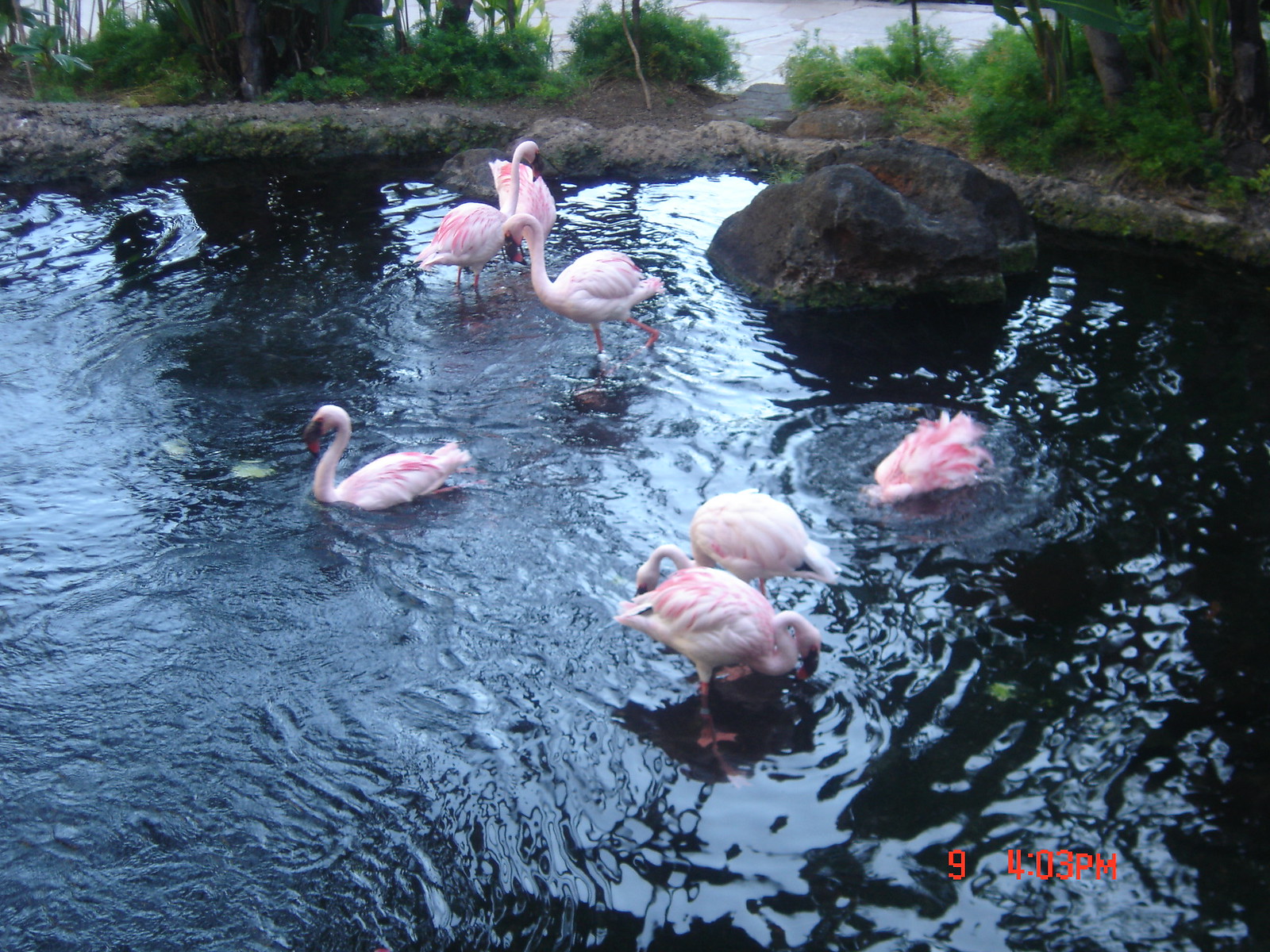This daytime photograph captures a group of six to seven pink flamingos in a large, man-made pond with dark blue water. The pond seems to be part of an outdoor habitat, likely an enclosure designed to replicate their natural environment. A prominent rock rests on the water surface toward the top right of the image, while the background features an island with a rocky base and lush greenery, including bushes and trees.

The flamingos are spread across the middle and foreground of the image, engaged in various activities. In the center, three flamingos stand, their heads dipped into the water, possibly searching for food. To the right, one flamingo is swimming with its neck elegantly arched, while another has only its tail visible above the water, surrounded by small bubbles, indicating it is diving.

The flamingos stand out with their white and pink feathers, long necks, and legs. They have black heads with black beaks, and the tips of their beaks are orange. The bottom right corner of the photograph features red text displaying the time "9 4 03 p.m," suggesting it was taken with a camera.